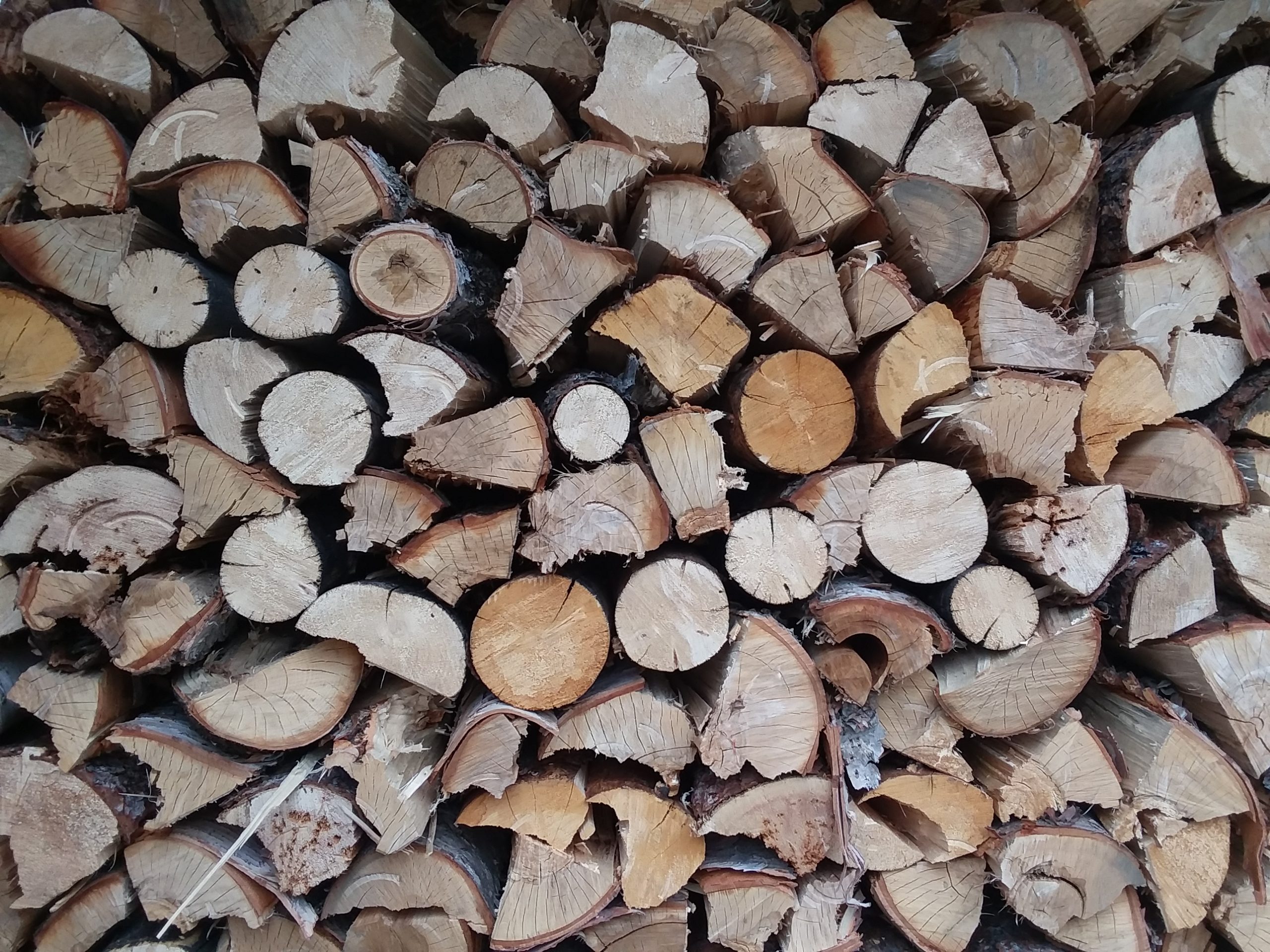The image displays a large, meticulous stack of firewood viewed from the side, filling the entire square frame. The wood pieces are arranged in multiple rows, creating a pattern-like appearance with various shapes and sizes—ranging from circular and triangular to random forms. The logs exhibit a range of colors: light tan with vertical cracks, dark brown layers, and even orangey to medium-tone browns. The outer layers of the wood vary too, with some sporting gray bark that's slightly peeled or turned up. Interspersed among the pieces are visible rings from where the logs were cut, and black spaces separating the chunks. Overall, the wood appears dry and cracked, highlighting the textures and characteristics of each piece.